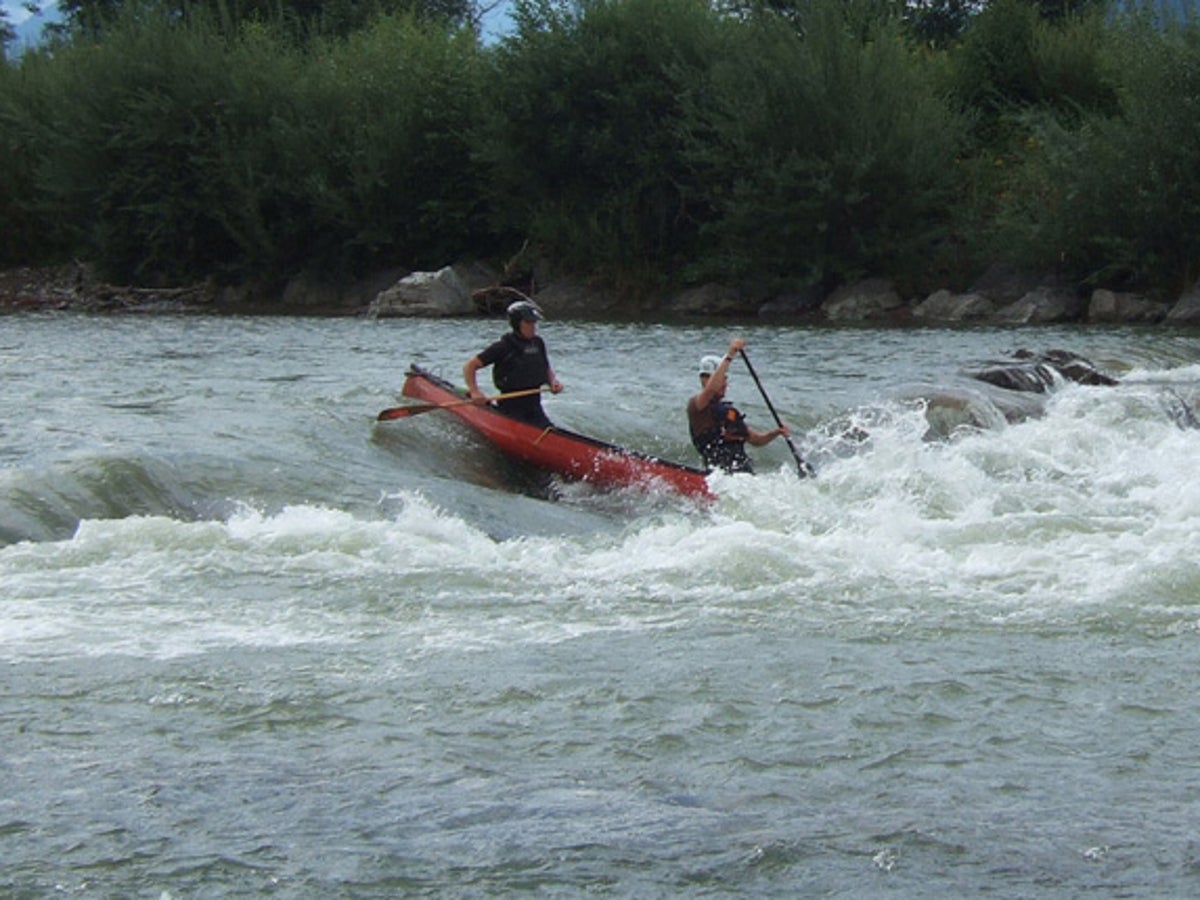The photograph captures a dramatic moment with two men navigating treacherous rapids in a red canoe with a black outline. Positioned at the center of the image, the canoe teeters over the edge from a higher point to a lower height, angled steeply with its bow pointing downward into rough, white-capped waters. The turbulent river churns around hidden boulders, creating a challenging terrain for the paddlers. Both men are dressed in black; the rear paddler wears a black helmet and holds his oar extended over the right side of the canoe, while the front paddler, donning a white helmet, dips his oar into the water on the left. The surrounding environment features a riverbank lined with a mix of evergreen trees and shrubby green vegetation that directly abuts rocky shores. The overcast conditions lend a grey, cold appearance to the river, enhancing the sense of danger and difficulty of this outdoor adventure.